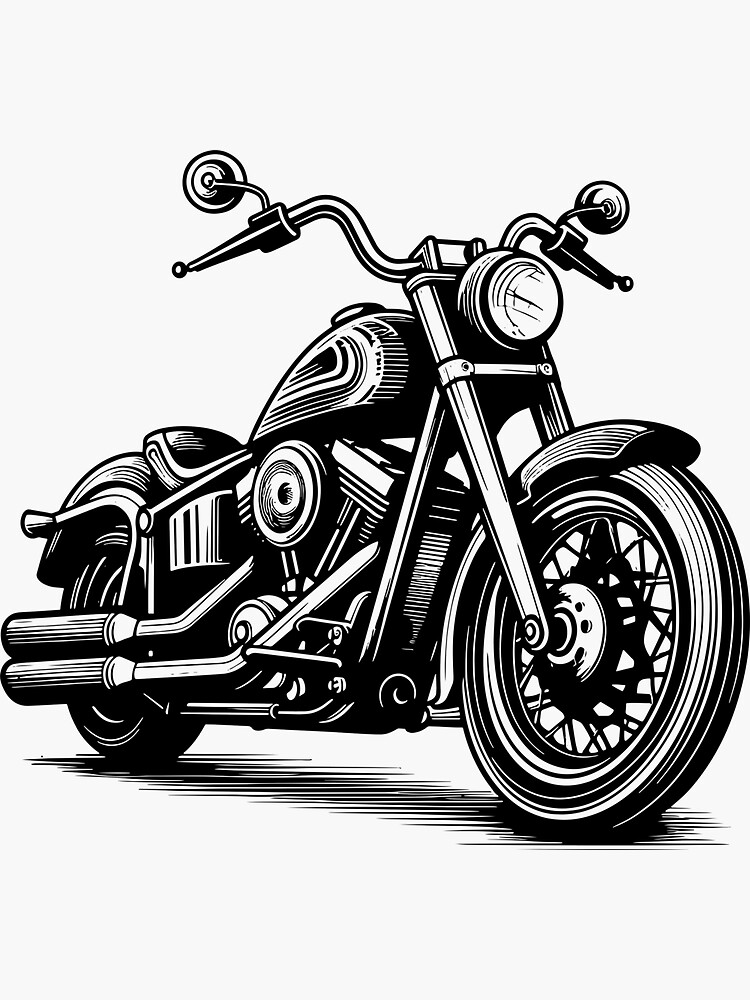This detailed image depicts a black and white drawing of a motorcycle, rendered in a style that resembles an animation or sketch, potentially akin to cartoon art. The overall image is vertically rectangular without a border, set against a light gray or white background. The motorcycle is oriented facing right, with a slight angle towards the viewer. 

The motorcycle features curved handlebars fitted with small round rearview mirrors and a prominent round headlight at the front. The dual exhaust pipes are visible on the left-hand side, with vertical black lines marking the ends. The bike includes a solid black leather seat, sitting above a teardrop-shaped gas tank with black and white accents. Both the front and rear wheels have curved fenders and black rims accented with white lines through and black tires with white sides.

Underneath the motorcycle, there's some black shading suggesting a light shadow. The engine is clearly visible below the seat, adding to the intricate details of this drawing. With no people, animals, or artist's signature present, this piece stands out as a meticulously crafted black and white depiction of a lone motorcycle.